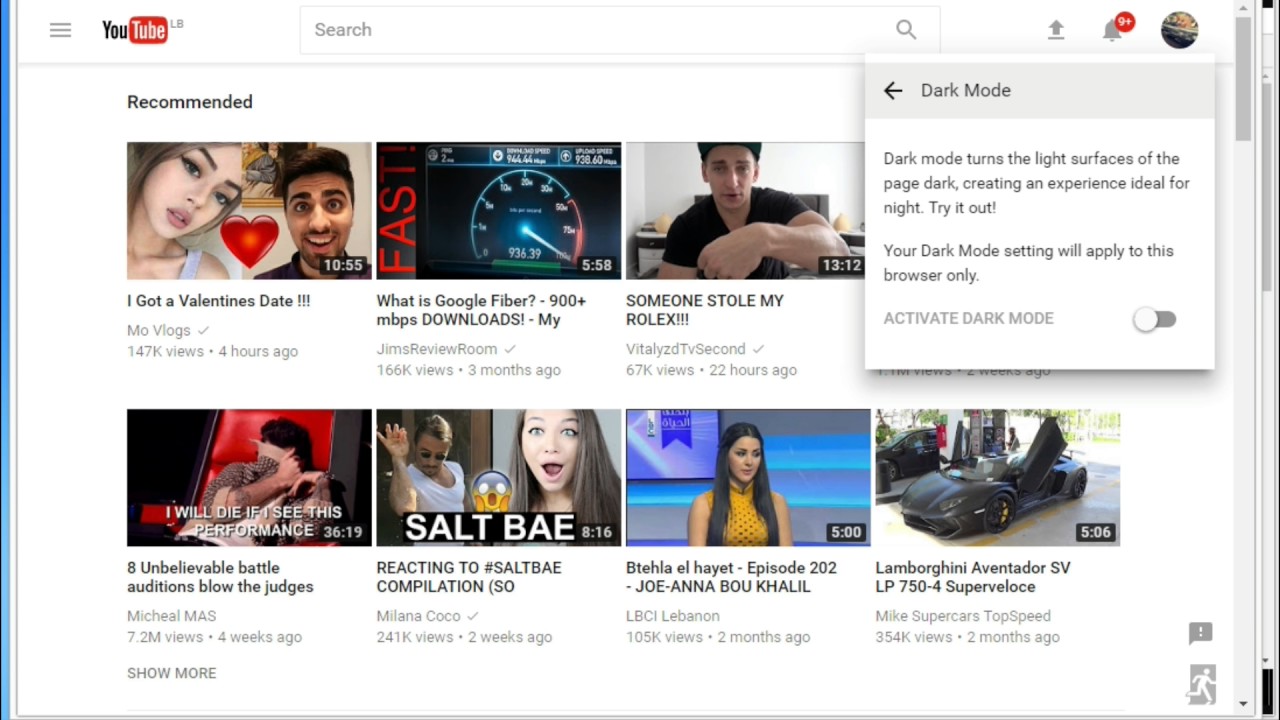The image showcases the YouTube homepage featuring recommended videos. There are two rows of video thumbnails, with four videos in each row, making a total of eight recommendations displayed prominently. The interface is in light mode, with a white background that highlights the content. 

At the top-right corner of the screen, there is a dark mode overlay box partially obscuring the fourth video in the top row. This box contains information about dark mode and options for toggling the feature on or off. The YouTube logo is positioned in the top left corner, flanked by a profile icon, a bell notification icon, and a download button in the top right corner. 

Central to the header is the search bar, poised above the video thumbnails for easy access. Adjacent to the YouTube sign on the left are three gray horizontal lines representing a menu or settings option, adding to the navigation functionality of the page.